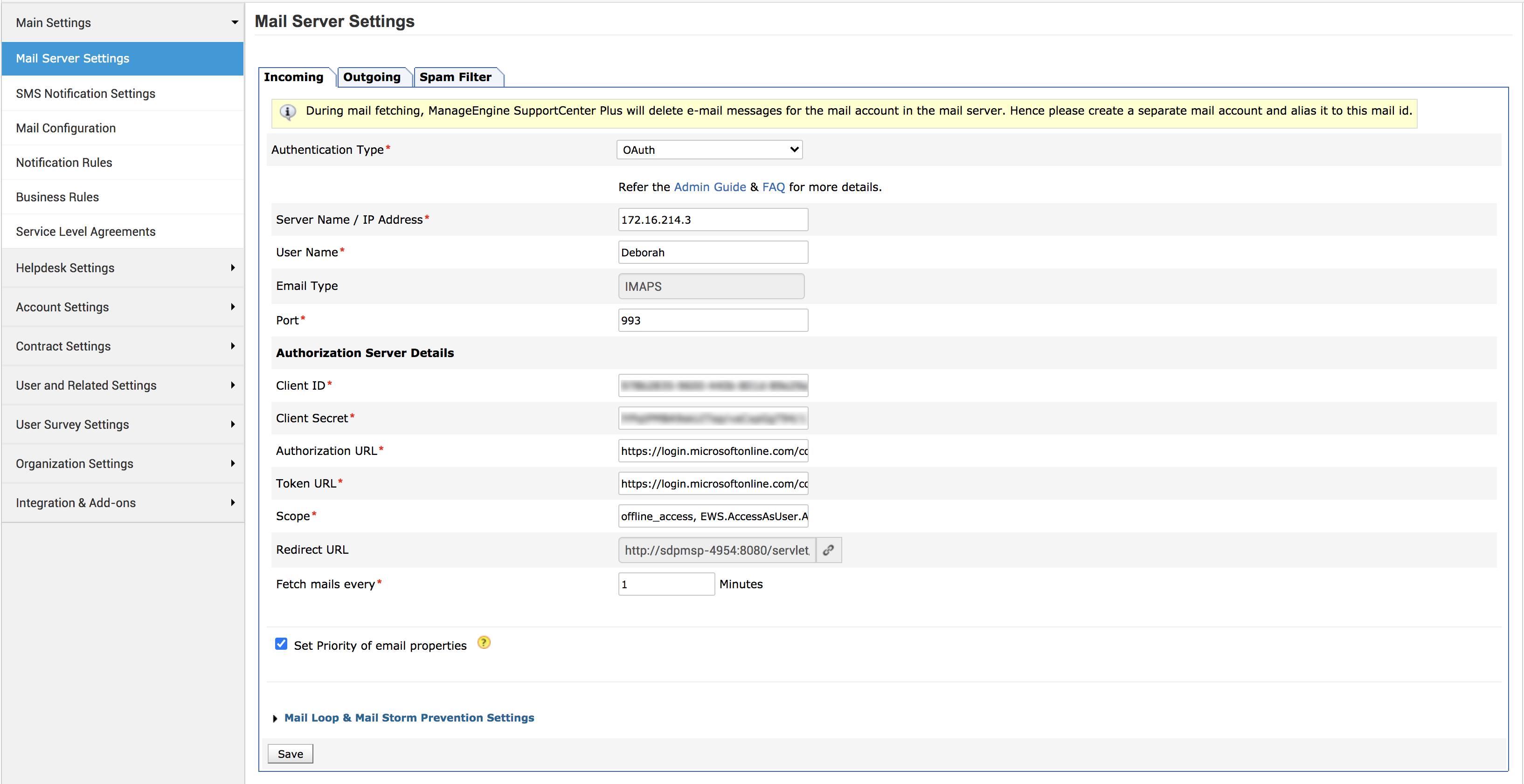A screenshot of a mail application on a smartphone, displaying the settings overview. In the upper left corner, there are options for "Main Settings" and "Mail Server Settings." To the right, tabs for "Incoming," "Outgoing," and "Spam Filter" are visible. Each tab has specific functionalities: the "Incoming" tab allows configuring rules for blocking or forwarding mail, the "Outgoing" tab manages settings for sent emails, and the "Spam Filter" tab provides customizations for filtering unwanted mail, including adding specific addresses and handling emails with attachments. This app, which is similar to but not exactly like Gmail, offers a comprehensive control panel for managing email settings, accessible both on a smartphone and potentially in a browser version.